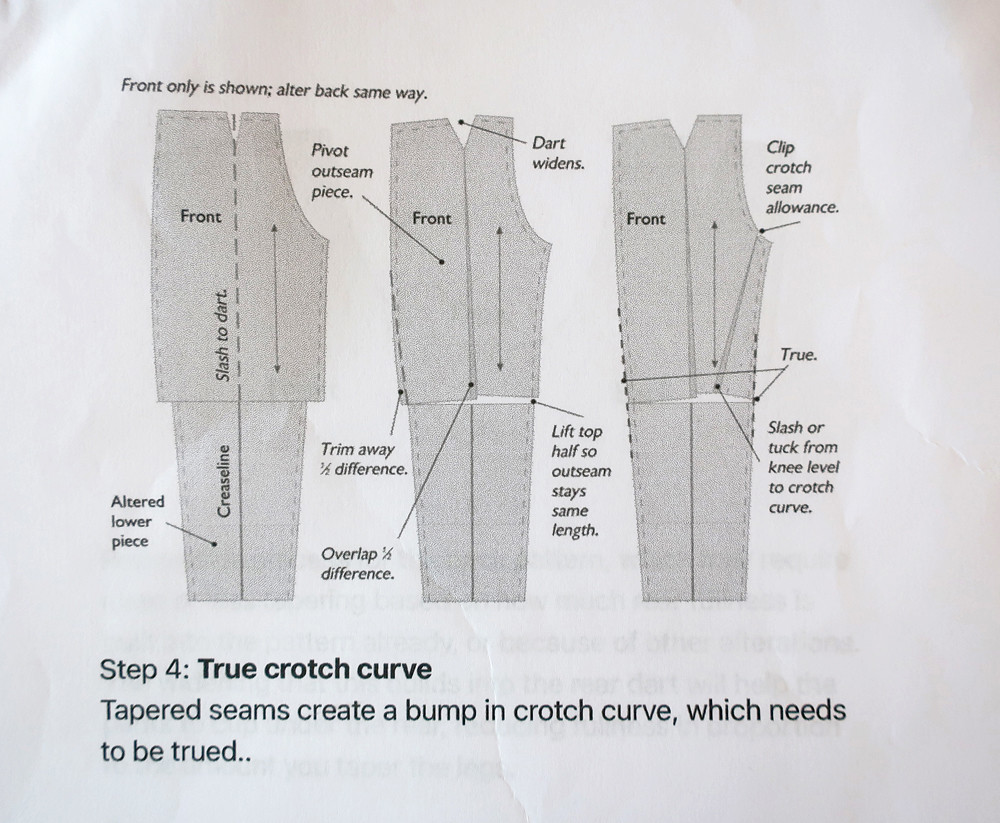This detailed image is a tailor's pattern and instruction sheet for altering a pair of pants, shown on a white sheet of paper. The top of the page states, "Front only shown, alter back the same way." There are three diagrams labeled "front" from left to right, each annotated with detailed instructions and arrows pointing to specific areas of the material. 

On the left diagram, notes include "altered lower piece" and "crease line." The center diagram instructs to "trim away one-half difference" and "overlap one-half difference," indicating changes near the midpoint of the piece, alongside guidance to "lift the top half so outseam stays the same length" and "dart widens."

The right diagram is focused on the crotch area with advisories like "clip crotch seam allowance" and "stash or tuck from knee level to crotch curve." Below these diagrams, emphasized in bold, is "Step 4: True crotch curve." The note further explains, "Tapered seams create a bump in crotch curve, which needs to be trued."

The instructions are meant to guide the tailor on how to fold, trim, and sew the fabric correctly, ensuring the proper fit and shape of the pants. The sheet appears to be a scan, as text from the reverse side is faintly visible.